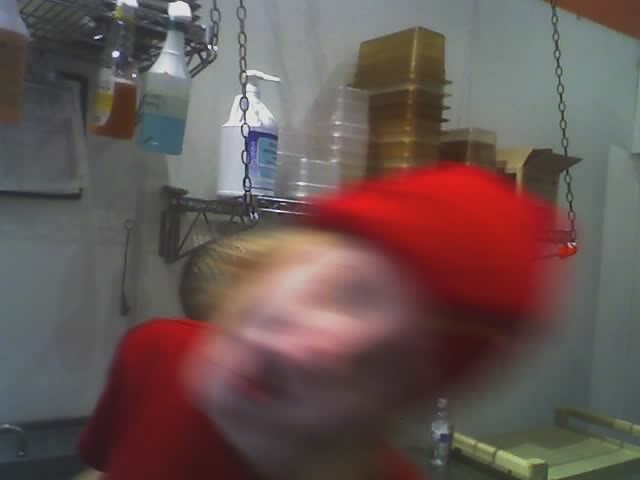In this blurred, color photograph, a person, possibly male, is in the foreground. They are wearing a red short-sleeved shirt and a red cap, with their blonde hair visible. The person's body is tilting to their left as they appear to look at the camera. Their face, though blurred, reveals red-pinkish lips.

The setting appears to be a kitchen, accentuated by a variety of visible details. On the gray wall behind the person, there are various shelves. One prominent shelf hangs with stainless steel chains and contains a large white pump bottle with a blue label, stacks of clear plastic empty containers, and some golden-hued plastic containers. Another shelf, a stainless steel wire one, is mounted in the upper left and has two labeled spray bottles: one with clear blue liquid and the other with a gold liquid. A white bin is also present on the wall.

Below the hanging shelf, there's a green cart or storage area with a water bottle placed next to it. Additionally, there is a plastic tray near the bottom right corner. In the distant background, a stainless steel sink with a visible faucet and a black cart add to the functional aesthetic of what seems to be a fast-food restaurant or a similar establishment.